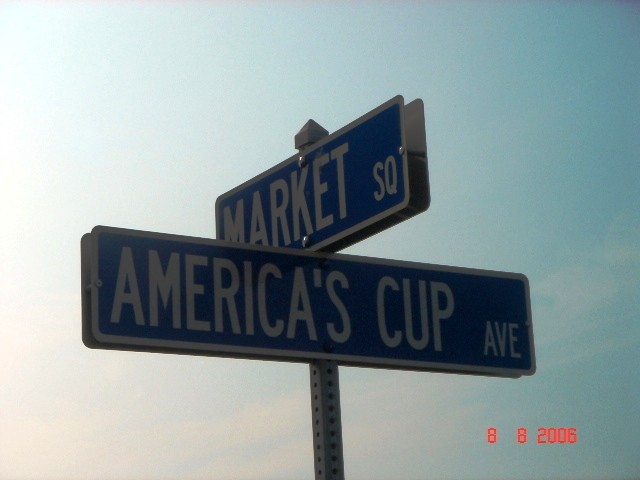The photograph captures an upward perspective of intersecting street signs against a backdrop of a clear daytime sky. The signs, which are blue with white lettering, prominently display "America's Cup Avenue" running horizontally from left to right. Diagonally opposite, angling from right to left, the sign reads "Market Square." A date, marked in red, is visible in the bottom right-hand corner of the image, stating "8 8 2006."